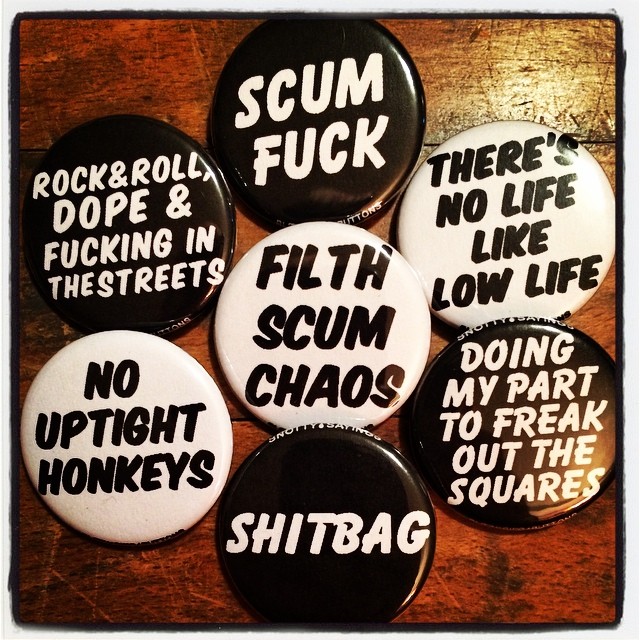The image depicts a collection of seven black and white clip-on buttons, arranged in a circular pattern on a dark, heavily scratched wooden tabletop. The button in the center has a white background with the message "Filth, Scum, Chaos" in black text. Surrounding it in a clock-like formation are the following buttons, starting from the top:

1. A black button with white text that reads "Scumfuck."
2. A white button with black text bearing the phrase "There's No Life Like Low Life."
3. A black button with white text that says "Doing My Part to Freak Out the Squares."
4. A black button with white text that simply states "Shitbag."
5. A white button with black text that proclaims "No Uptight Honkies."
6. A black button with white text declaring "Rock and Roll, Dope and Fuckin' in the Streets."
 
The buttons are described as humorous, albeit possibly vulgar, and are arranged to create a visual similar to a flower, with each one radiating out from the central button.